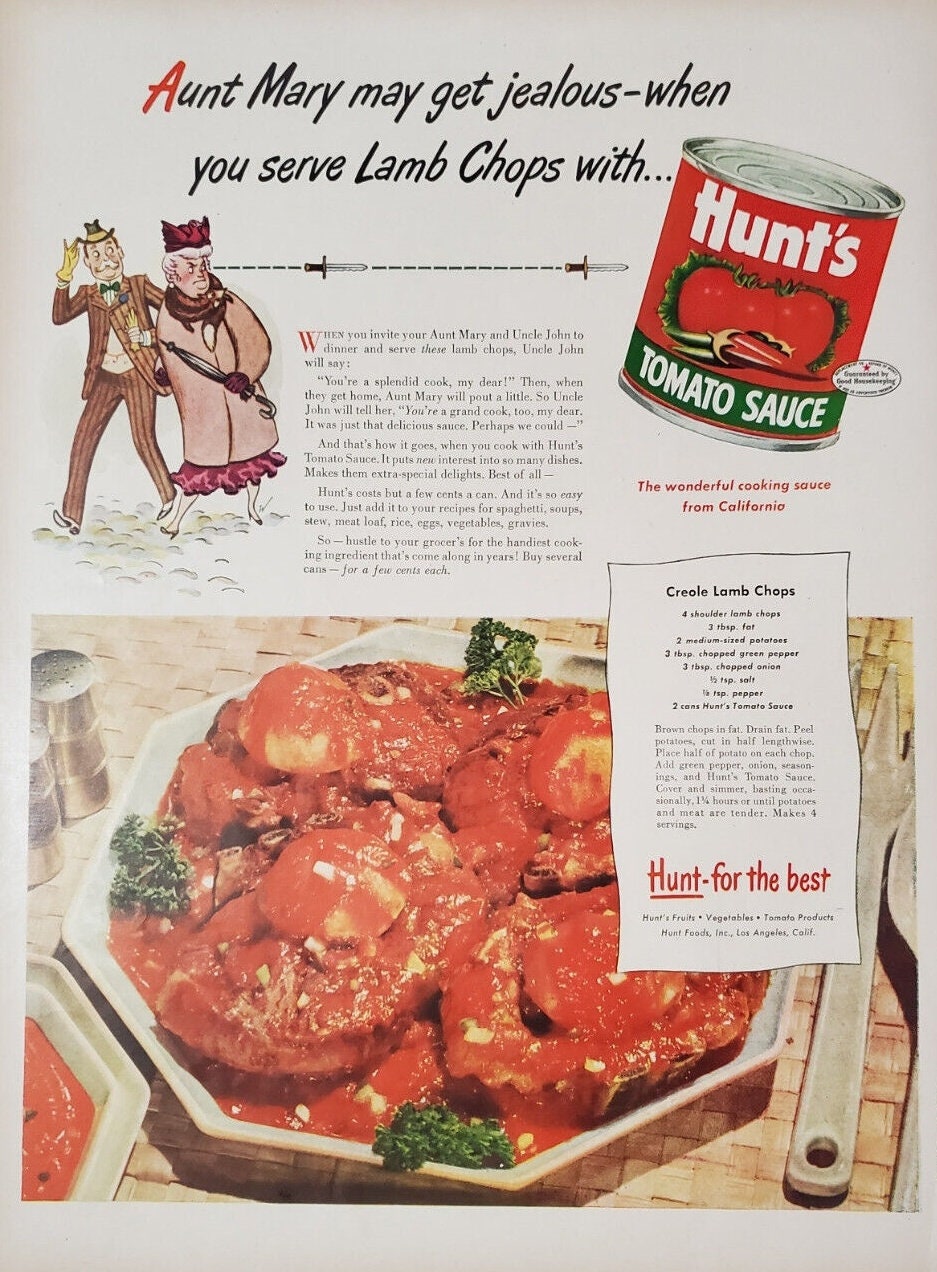This is a vintage advertisement featuring Hunt's tomato sauce, accompanied by a detailed recipe for Creole lamb chops. In the upper right-hand corner, the centerpiece is a red can of Hunt's tomato sauce. The headline reads, "Aunt Mary may get jealous when you serve flame chops." To the left, a charming cartoon shows a woman in a pink dress and long coat, holding an umbrella and glaring jealously towards the can, with her husband in a brown pinstriped suit beside her. The narrative promises that when you invite Aunt Mary and Uncle John for dinner and serve them these delectable lamb chops, Uncle John will commend your cooking, causing Aunt Mary to pout even as she reluctantly admits it was a delicious meal. Below, there's an appetizing image of the lamb chops in rich, red sauce, presented on a hexagonal plate with a fork and spoon on the side, and another dish partially visible on the left. Overlapping this picture is a cut-out-style recipe for Creole lamb chops, framed with the tagline at the bottom, "Hunt for the best." This advertisement highlights the versatility and affordability of Hunt's tomato sauce, perfect for enhancing various dishes with just a few cents per can.